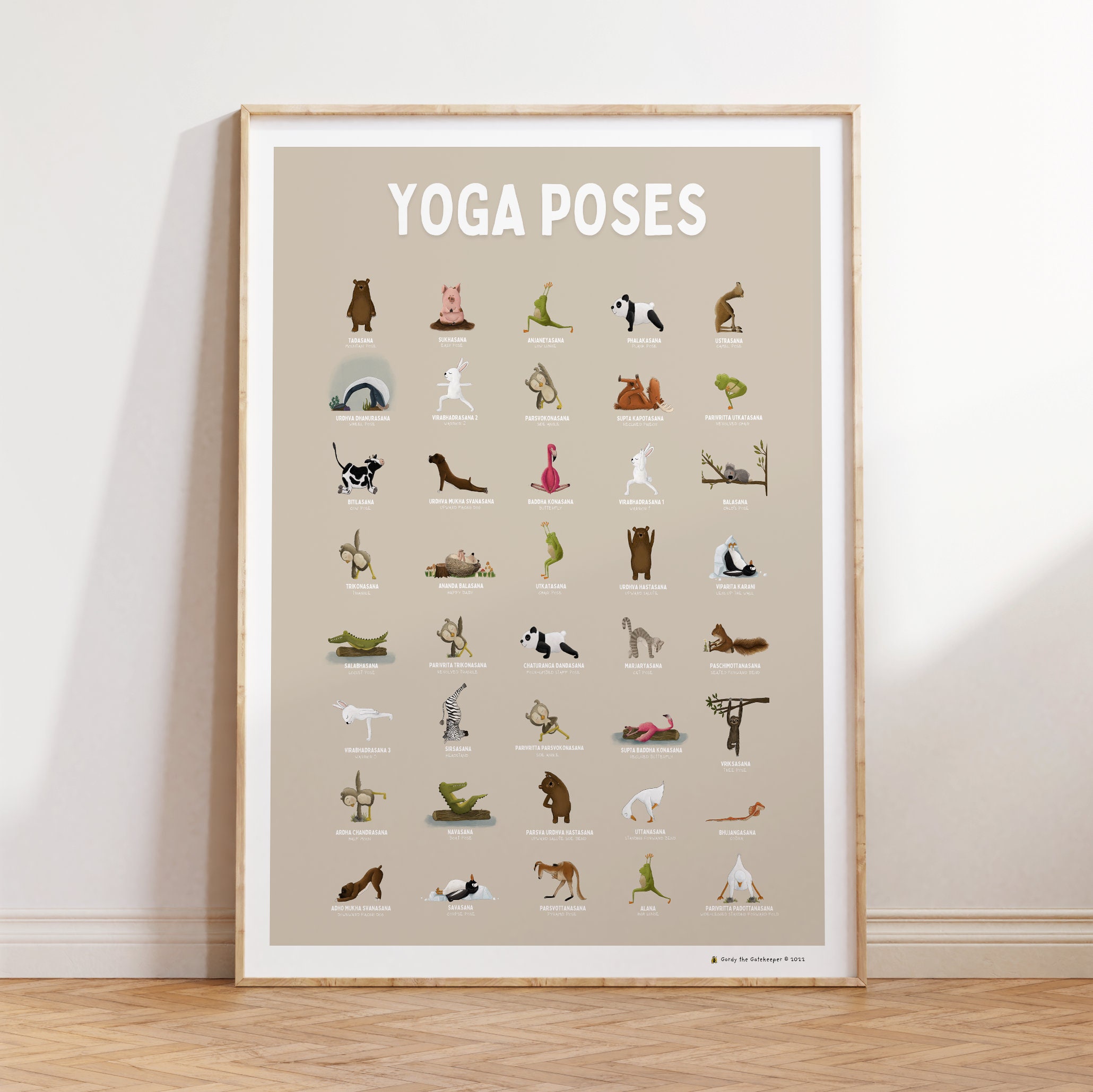The image depicts a whimsically illustrated poster, elegantly framed with a light brown border and set against a white wall with off-white trim. The poster rests on a brown, zigzag-patterned wooden floor. Dominating the top center of the poster, the phrase "YOGA POSES" is prominently displayed in all capital white text. The poster comprises 40 different yoga poses, each amusingly demonstrated by various animals. These animal illustrations, set against a light brown background, include bears, pigs, frogs, pandas, kangaroos, lemurs, squirrels, koalas, flamingos, alligators, and possibly zebras or leopards. The animals are depicted in assorted colors such as brown, pink, green, black, and white. Each pose is accompanied by white text beneath the animals, though it is too small to be deciphered. Similarly, some black text in the lower right corner of the poster remains illegible. The collection of various animals in whimsical yoga positions provides a playful and engaging visual experience.